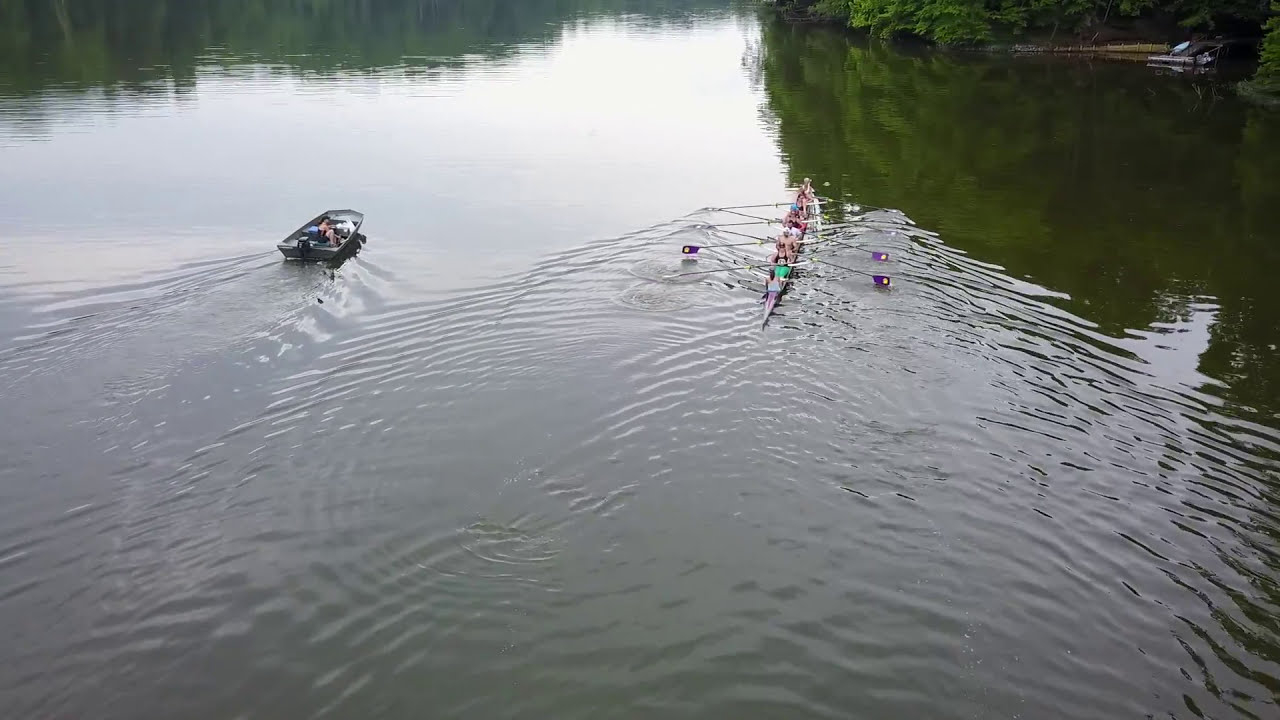The image captures a serene, expansive body of water during the day, featuring a rowing scene. In the center-right of the photo, four rowers propel a long rowboat using purple oars. Off to the left is a motorboat, appearing to keep pace with the rowers. Ripples trailing behind both vessels suggest they are in motion. The water, reflecting the surrounding environment, appears brownish due to the reflected light from trees, whose actual presence is more visible at the top edge of the photograph. Additionally, in the upper right corner, there's a small dock or structure. The scene, devoid of any text, is bathed in natural colors including green, white, gray, pink, light blue, tan, and black, perfectly capturing an outdoor waterscape.